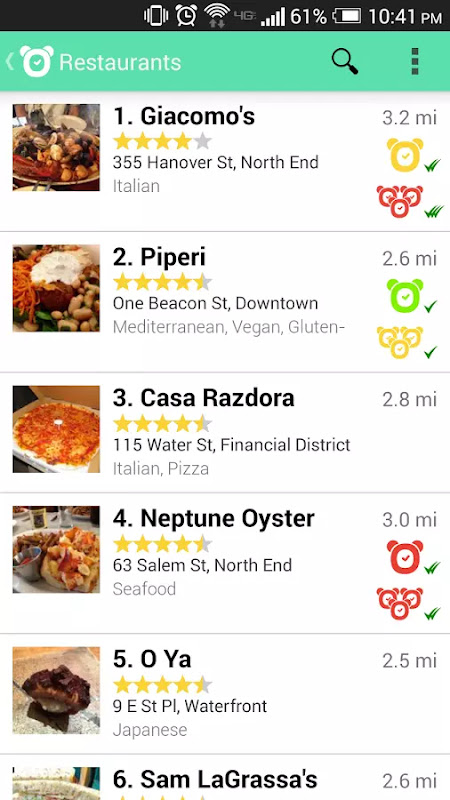The phone screenshot shows a detailed display of various smartphone indicators and a list of nearby restaurants. At the top of the screen, the time is shown as 10:41 PM in white text against a black background. Next to the time, the battery indicator shows 78% charge. Below the battery icon, the text indicates 61% battery, which appears incorrect. The phone has full reception bars in white and displays "4G" in gray. Additional icons include a white Wi-Fi symbol, an alarm clock, and a vibrating phone icon.

Below these indicators, a green and white background features a leftward-pointing arrow and a white clock icon. The text "Restaurants" appears in white with a black magnifying glass next to it, followed by a list of restaurant names and ratings, each in a black box:

1. **Giamo's** - 4 stars.
2. **Pipery** - 4.5 stars.
3. **Casa Rosa Dora** - 4.5 stars.
4. **Neptune Oyster** - 4.5 stars.
5. **Oya** - 4.5 stars.
6. **Sam’s La Grassa** - distance not fully visible.

The displayed distances to the restaurants are 2.5, 3.2, 2.8, 2.6, and 3.2 miles away, respectively. The detail for Sam’s La Grassa is cut off, making it difficult to see the stars and the exact distance.